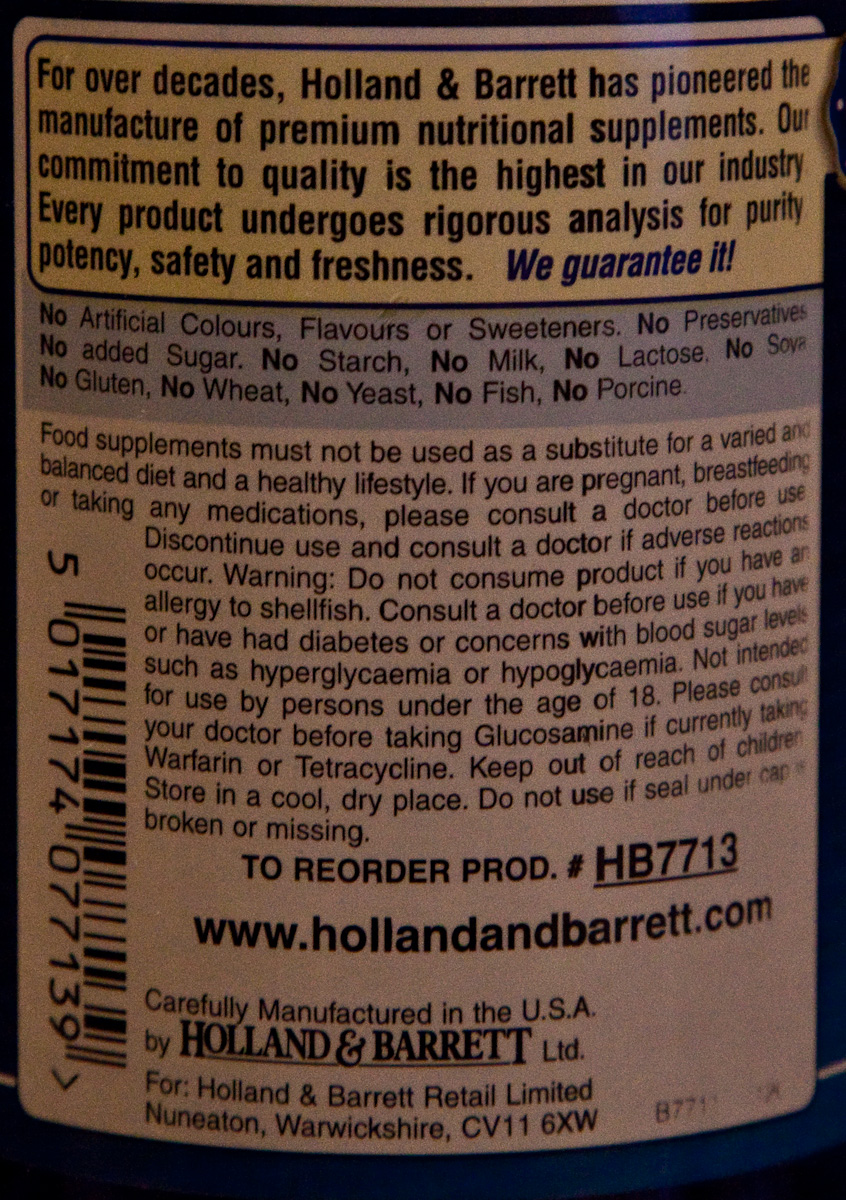This image is an extreme close-up of the back label of a nutritional supplement bottle by Holland & Barrett. The label, on a white background with a blue strip in the middle, prominently features black lettering. Starting at the top, the label details the brand’s history, stating, "For over decades, Holland & Barrett has pioneered the manufacture of premium nutritional supplements." It emphasizes their commitment to quality, noting that every product undergoes rigorous analysis for purity, potency, safety, and freshness, and guarantees these standards in italics.

The label also lists what the supplement does not contain: no artificial colors, flavors, sweeteners, preservatives, added sugar, starch, milk, lactose, gluten, wheat, yeast, fish, or porcine. Additionally, it includes a disclaimer that supplements should not be used as a substitute for a varied and balanced diet and advises consulting a doctor before use, especially if pregnant or breastfeeding.

On the left side, a barcode is visible, along with the reorder product number and the website, hollandandbarrett.com. The label notes that the product is carefully manufactured in the USA for Holland & Barrett Retail Limited, located in Nuneaton, Warwickshire, UK, highlighting the British origin despite the American manufacture.